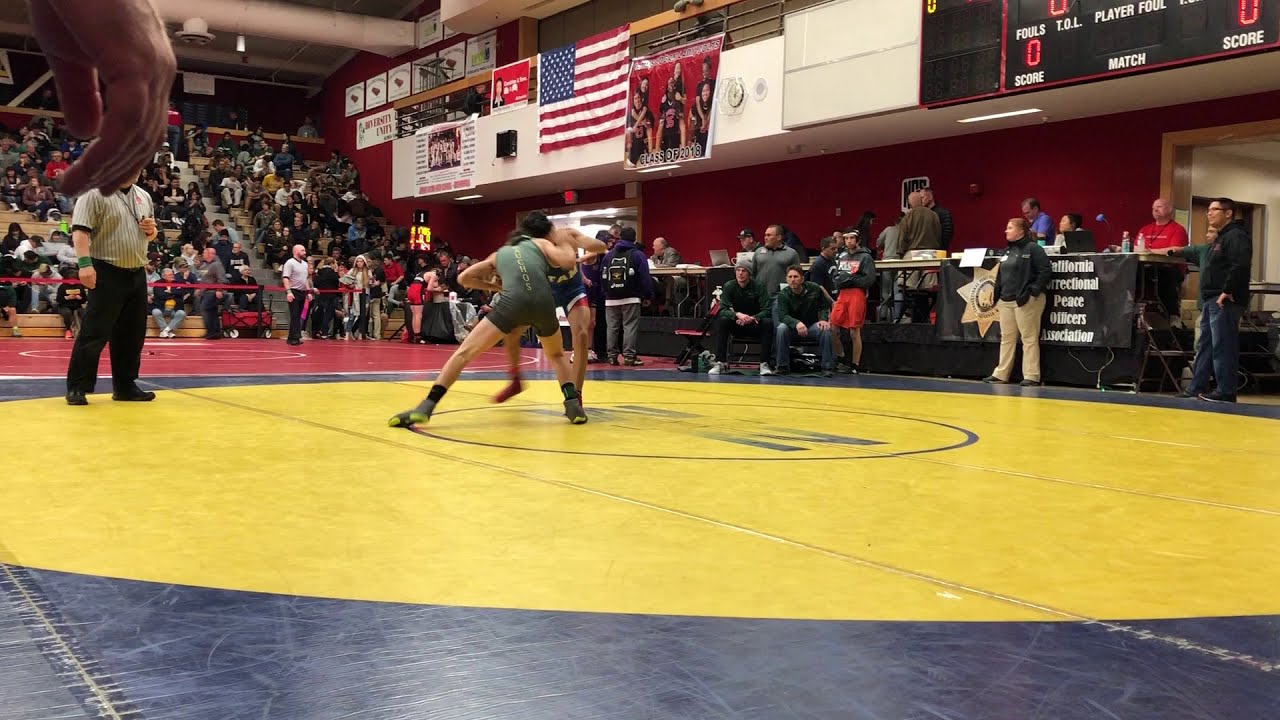In this detailed photograph of a high school wrestling tournament, the scene captures two white wrestlers intensely engaged on a yellow and blue mat. One wrestler is clad in a green outfit, while the other sports a dark blue uniform. They are the focal point, positioned centrally but somewhat distant from the camera's perspective. To the left, the referee stands in his black pants and striped black-and-white shirt, holding a whistle. Notably, his head is obscured by a photobombing hand that appears close-up in the top left corner of the image, cropping off just below the wrist.

Surrounding the wrestlers, a row of folding tables is visible on the right side, populated by announcers and support staff. Behind the action, the background features bleachers filled with spectators, with only a few empty seats scattered amongst the crowd. The upper portion of the frame reveals part of the venue's wall and the edge of a scoreboard, hinting at the spacious environment hosting the event.